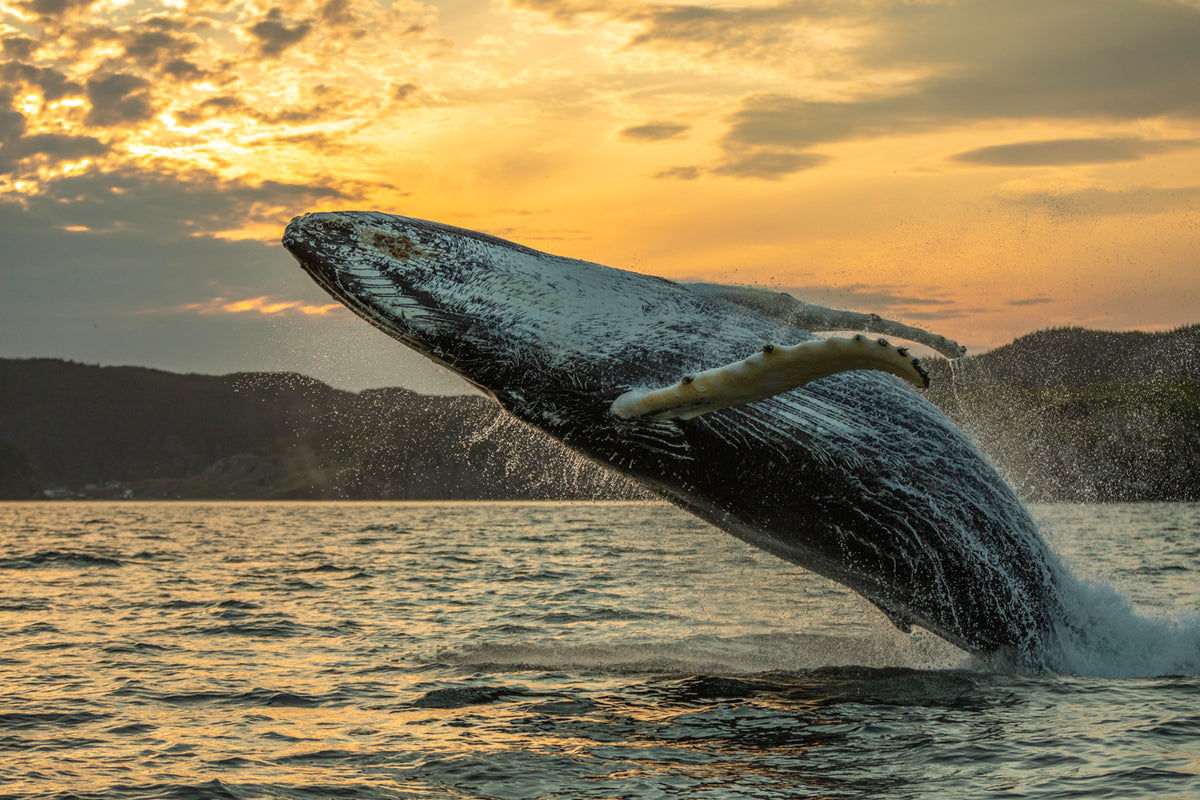In this stunning photograph, a massive humpback whale is captured in the midst of a dramatic breach, leaping powerfully out of the ocean. The whale is upside down at the acme of its leap, with its tail still partially immersed in the turbulent, foamy water below. Its body is a striking dark blackish-gray, complemented by a whitish underbelly adorned with distinctive white marks. The fins of the whale exhibit a light beige hue.

The scene unfolds against a breathtaking twilight backdrop, with the sun having just set. The horizon glows with a sherbet orange light that bathes the ocean and the whale in a warm, golden hue. The twilight sky is speckled with gray clouds, each one backlit majestically by the waning sunlight. In the distance, a rugged, hilly shoreline with imposing mountainous terrain frames the composition, adding depth and intrigue to the image, which combines the serene blue of the water with the fiery oranges of the setting sun.